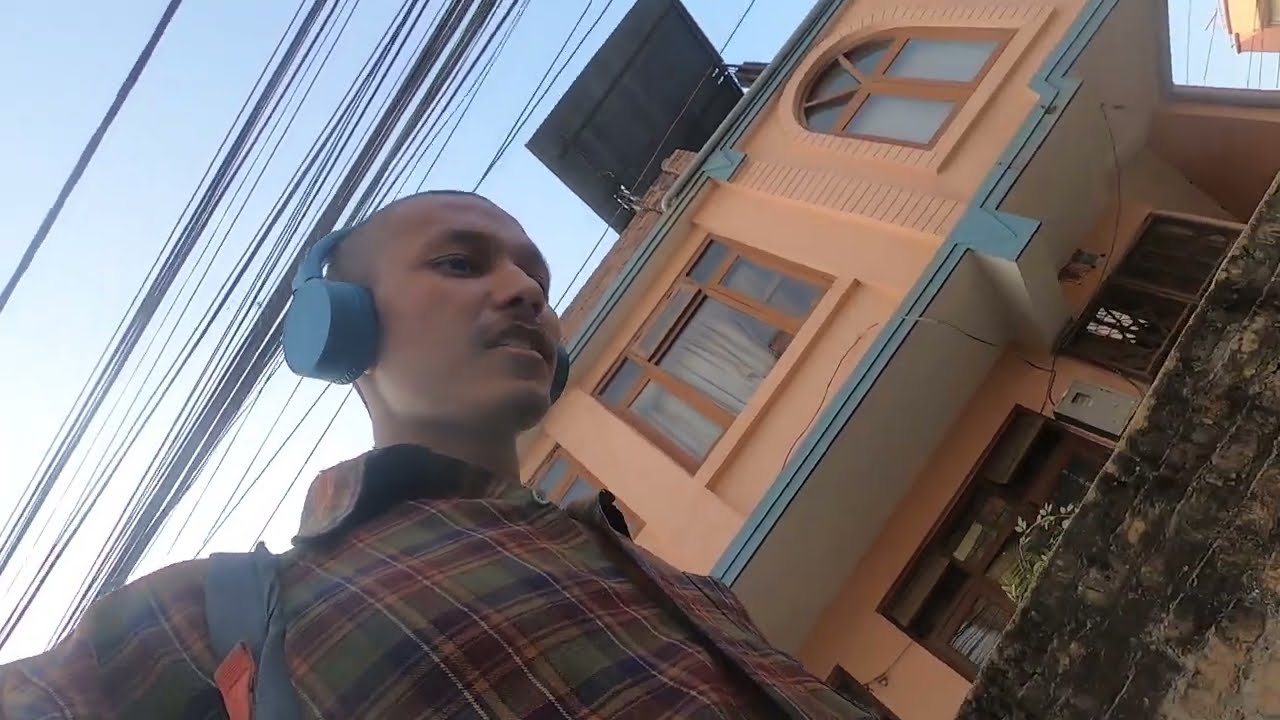The photograph captures a skewed, upward-looking perspective of a tan-skinned bald man with Asian features, who appears to be standing against a two-story, stucco building painted in a terracotta or orangish-pink hue with light blue accents. He is wearing light blue headphones and a plaid shirt in green and dark red, complemented by a gray backpack strap with orange detailing. The image is tilted about 45 degrees to the right, as if taken from ground level. Surrounding him, the scene includes multiple electrical wires crossing the sky, which is a clear light blue with some white clouds. The building features brown windows adorned with plants or vines and has an algae-covered stone wall at the base.